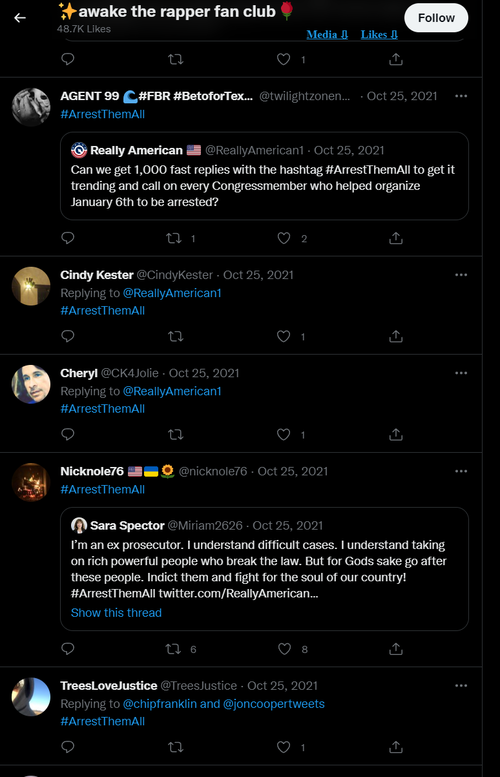The image depicts a Twitter page with a black background. At the top left corner, there is a white arrow pointing left. To the right, three yellow stars are followed by the text "Awake the Rapper Fan Club" in white, alongside a red rose icon. Below that, in white text, are the words "Follow" and "48.7 likes."

A blue tab labeled "Media Analytics" is present, with "Agent 99" written in white next to it. There are additional symbols and text, including a wave icon, a pound sign, and the phrase "yard pound BET B24" followed by ellipses. The text "@twilightzone" appears, and "October 25, 2001" is noted in blue, accompanied by the phrase "arrest them all."

The main focus of the page is a tweet replying to "Really American" who posted on October 25, 2001, calling for "1,000 fast replies with #arrestthemall to ensure every crime-fixing member involved in the NY6 incident is brought to justice". This tweet is being responded to by "Cindy Hester," replying to "@American1" with "#arrestthemall" and "Cheryl" who is "@ck4joey". Both tweets are timestamped "October 25, 2001" and include similar calls to action with the hashtag #arrestthemall. Another user, "Nick No 76," also joins in, replying on the same date with "@arrestthemall".